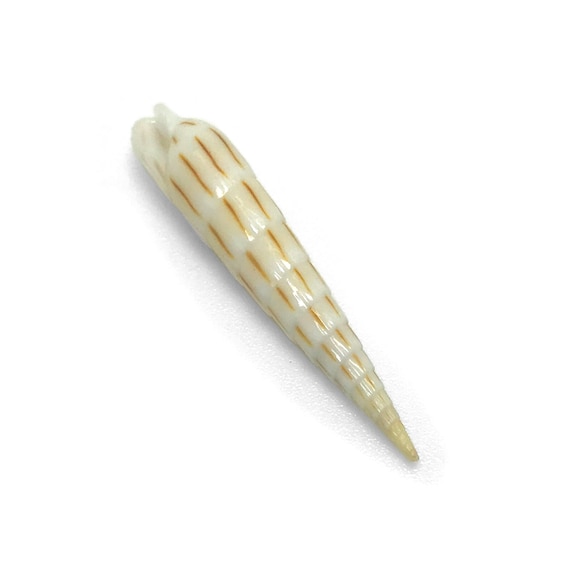The image features a close-up capture of a single seashell against a plain white background, filling the entire frame. The seashell, resembling a conch or snail shell, is positioned diagonally, extending from the upper left corner to the lower right corner of the image. It exhibits a spiral pattern, winding round and round, creating a shape that is sharp, spear-like, and tapering to a point at the bottom right corner. The shell's ivory base is adorned with distinct brown striations that run vertically when viewed in alignment with its diagonal orientation. The shell, approximately four inches in size, has a rounded upper part with a small stem-like projection and narrows significantly towards the bottom, giving it a screw or carrot-like appearance.